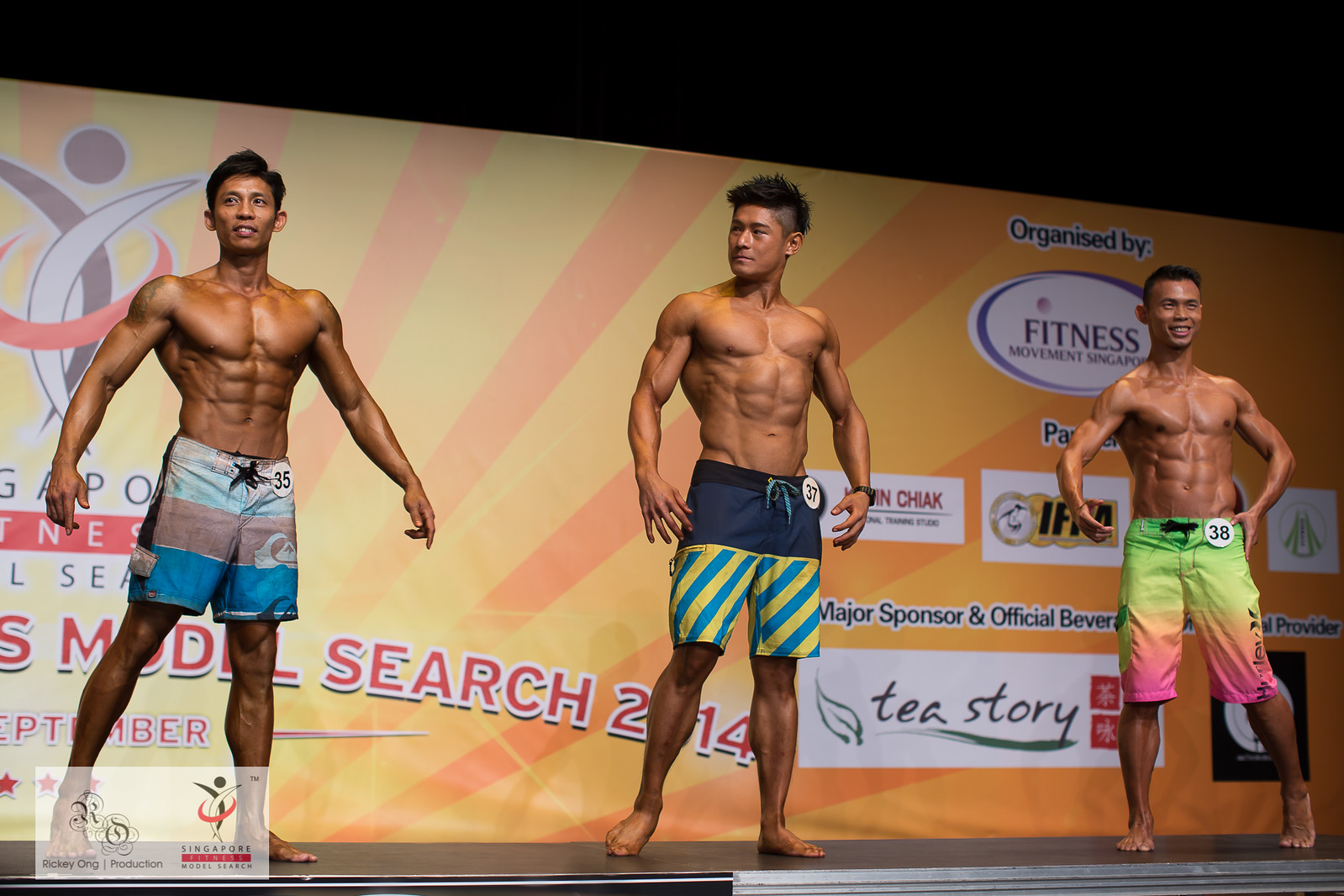The image depicts a vibrant moment from the "Model Search 2014" bodybuilding competition, featuring three muscular contestants posing confidently on stage. Each man is shirtless and barefoot, wearing knee-length swim trunks of varying designs. The contestant on the right stands out in his colorful swim trunks with green, yellow, orange, and pink hues, displaying a prominent six-pack while flexing. The man in the middle dons blue swim trunks with blue and yellow stripes on the bottom, highlighting his muscles in a less intense pose. On the left, the third competitor sports blue and gray striped trunks with a Quicksilver logo, striking a pose of his own.

They are positioned in front of an eye-catching banner that showcases a rising sun with alternating rays of golden orange, surrounded by numerous sponsor logos. Each contestant has a number displayed on the belt of their trunks; these numbers are 35, 47, and 48. The overall ambiance is rich with colors such as yellow, orange, green, purple, blue, black, brown, and white, enhancing the lively atmosphere of this competitive event.